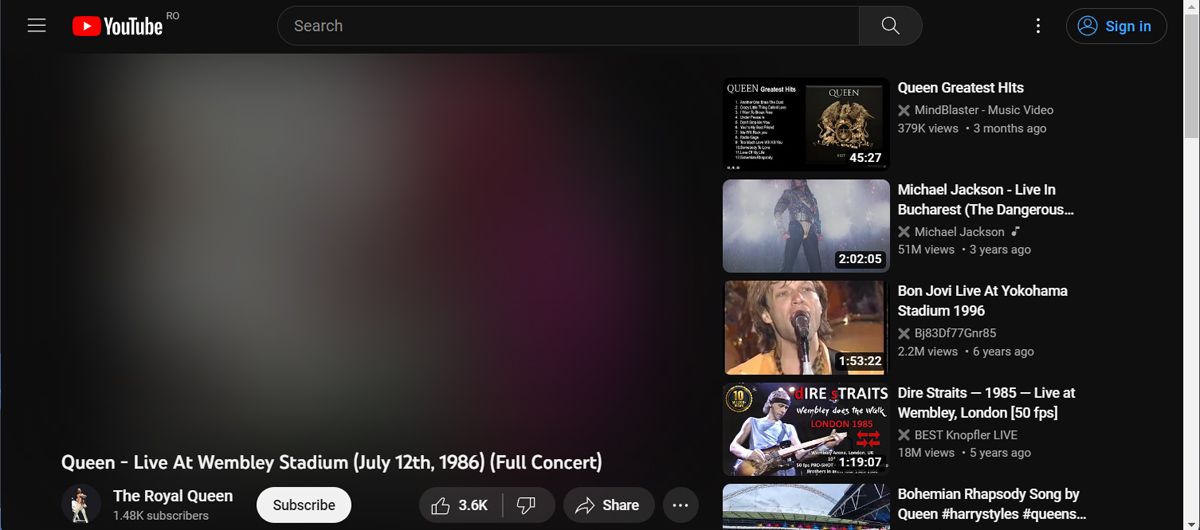The YouTube search page features a predominantly black background with a black banner at the top. On the top left, there is a three-line menu icon. Immediately to the right of this icon, the recognizable red YouTube logo with a white play arrow is displayed next to the white "YouTube" text. Above this text appears the letters "RO."

Central on the page, there is a search bar, and on the right end of the search bar, there's a three-dot menu icon. Further right in an oval shape is an icon resembling a generic profile picture, outlined in blue, followed by the text “Sign in” in blue.

Beneath the search bar, the content section of the page is predominantly black with some gray and purple hues. Spanning from the left side about three-quarters across the page, there is content displayed regarding a video titled "Queen - Live at Wembley Stadium," including the date and additional concert details. Below this, users have the options to like, share, and subscribe, with the subscribe option displayed in white.

To the right of the main video content, there is a list of four to five recommended videos. These include a variety of images and titles, primarily featuring content related to Queen. The top recommendation on the right is titled "Queen's Greatest Hits," followed by videos about Michael Jackson, Bon Jovi, Dire Straits, and "Bohemian Rhapsody" by Queen. This list includes timestamps and further information about each video, offering an assortment of music-related video recommendations.